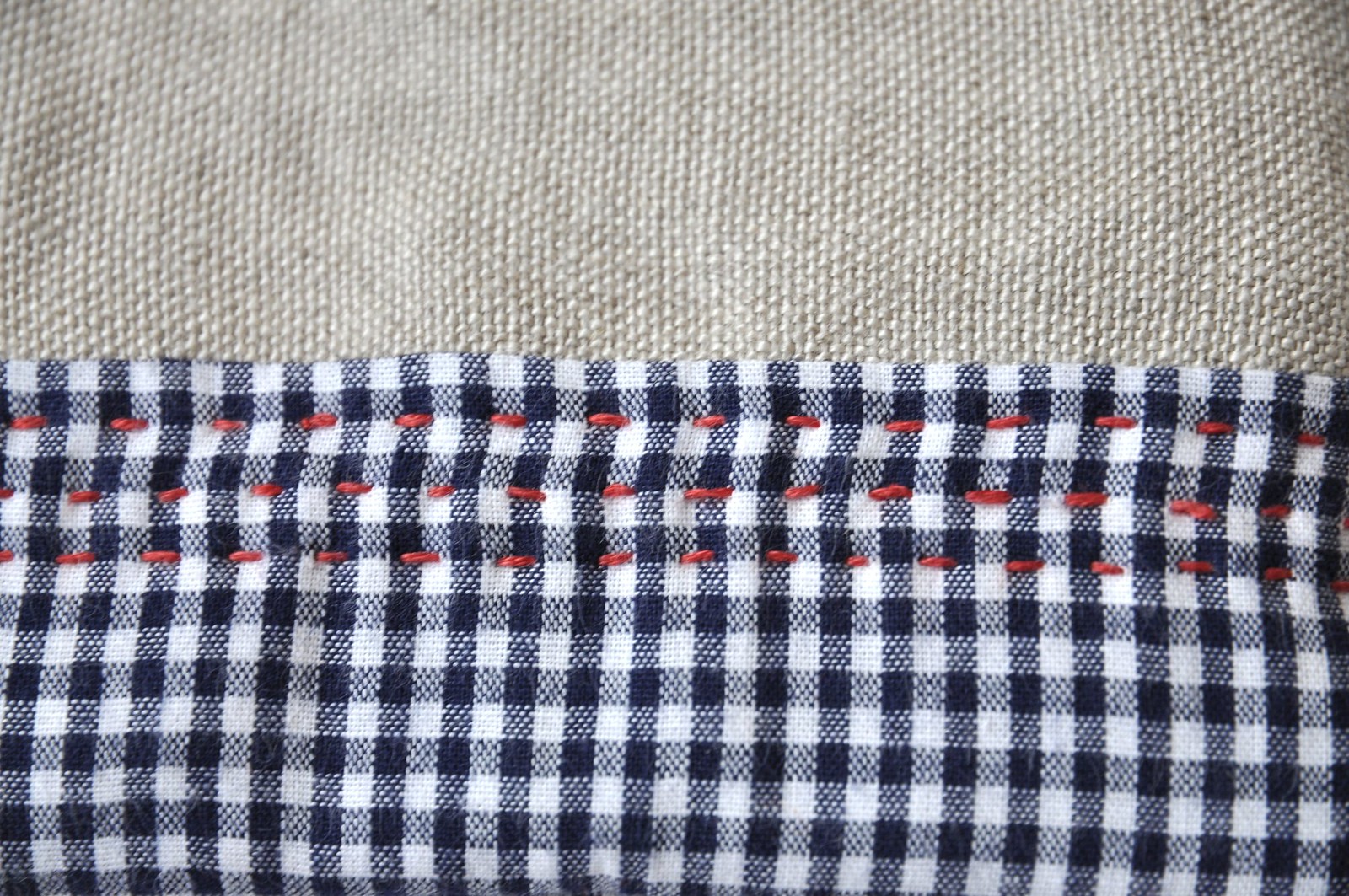The photograph is a detailed close-up of two distinct pieces of fabric stitched together with red thread. The top fabric resembles a thick, light tan wool or canvassy gray textured material, while the bottom fabric is characterized by a blue and white checkered, cotton-like pattern. The fabrics, differing in texture and color, appear mismatched and are connected by three rows of irregular, hand-stitched red stitches. Each visible row of stitches runs through both pieces of fabric at the center with the bottom row having 15 stitches, the middle row 14, and the top row 16. The stitching is uneven, indicative of handwork, with each stitch spaced approximately half an inch apart. The image is focused solely on these fabrics; there are no people, text, or other objects visible in the frame, and the background surface is not discernable. The overall appearance of the fabrics and stitching suggests they are aged and not of high quality, giving the scene a somewhat worn and unattractive look.